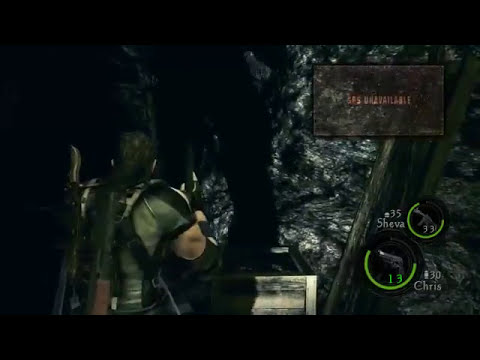In this dark and atmospheric screenshot from the video game Resident Evil 5, the main character, a robust male soldier wearing a short-sleeve green uniform, stands on the left-hand side of the screen, gazing down a narrow, dimly lit cavern or tunnel. His back is to the viewer, showcasing his well-built physique and brimmed with weaponry, including a large gun and possibly a knife or machete strapped to his back. In his right hand, he holds a pistol in a defensive stance, poised to confront whatever dangers lie ahead. Within the grayscale and green-hued environment, a wooden beam stretches upward along the left-hand side, and a wooden cart is situated directly in front of him, adding to the immersive setting. The right side of the screen features the game's user interface: a large block of text in red letters reads "SOS Unavailable," while concentric circles display the ammunition status for both the main character and a side character named Shiva. The top circle indicates "33" bullets with a total of "35" and the name Shiva, whereas the lower circle indicates "13" bullets out of "30" for the character Chris. Illuminating the enigmatic cave, silver and gray stones frame the scene, further enhancing the sense of foreboding and adventure.